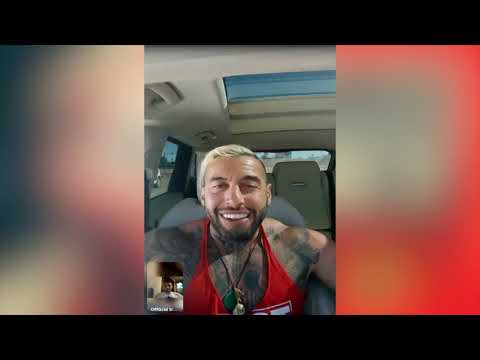In this color photograph, a muscular man wearing a red muscle shirt and a necklace takes a selfie while seated inside a car with a beige interior. His heavily tattooed arms, adorned with dark and unidentifiable designs, are clearly visible. The man has frosted platinum blonde hair and a scruffy beard and mustache, while a cheerful smile lights up his face. He appears to be on a video call, evidenced by a smaller inset image in the lower left corner showing another person, who may be wearing a white shirt, though the details aren't clear. The car's interior features a visible moonroof and views through the side and back windows. The photograph is set within a horizontal rectangular frame with dark borders on the top and bottom and a reddish-gray border on the sides. The main image is centered in a portrait orientation, inset against an enlarged, slightly blurred background of the same image, creating a layered effect.